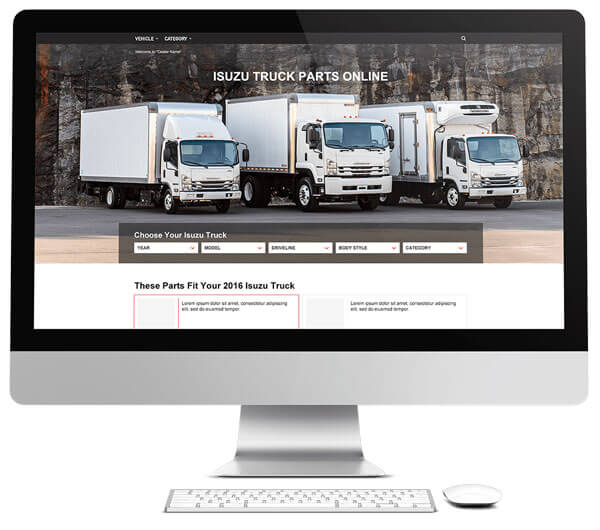The image is a screenshot of a computer monitor with a black bezel and a silver strip at the bottom, all situated on a sleek, shiny silver base. The monitor has a distinct bend where the base meets the screen, enhancing its modern, stylish design. In front of the monitor is a white keyboard with matching white keys and a small, white mouse placed to its right, all set against a pristine white background.

The screen displays a website featuring three large, white Isuzu trucks. At the top of the screen, white text reads, "Isuzu Truck Parts Online." Below this, there are dropdown menus and buttons labeled "Choose Your Isuzu Truck Year" and "Model," though this text appears blurry. Further down, the screen states, "These parts fit your 2016 Isuzu truck," indicating the specific model year that the website caters to.